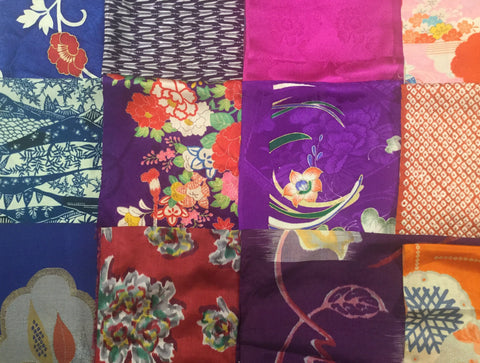This color photograph showcases a close-up of a vibrant quilt composed of evenly lined-up squares, each approximately 6 by 6 inches in area. The quilt features a total of 12 visible squares, each displaying a unique pattern. The predominant colors are rich shades of purple, orange, pink, and blue. Several squares boast floral designs, including one with a purple background adorned with an orange flower and another with a blue background featuring a red flower. There are also geometric patterns and a picturesque patch with a rough country scene. One square stands out with a solid fuchsia color, while another, located in the bottom left, has a dark blue background with a flame motif in the bottom right corner. The overall theme harmonizes plant and flower motifs with swirling shapes, creating a vibrant and diverse tapestry.